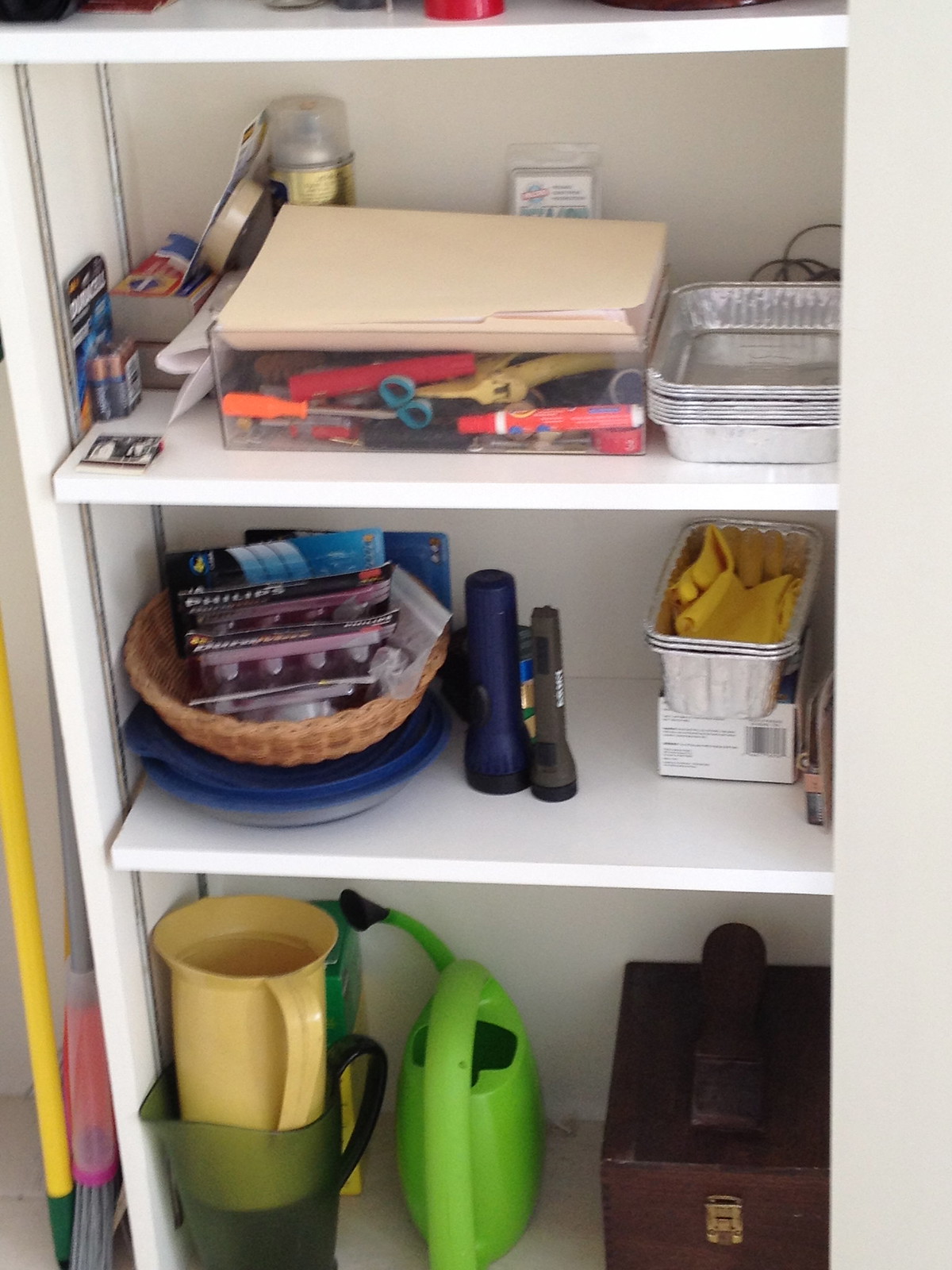A well-organized pantry nook features three wooden shelves stocked with household essentials. On the bottom shelf, a green plant watering can and two handheld pitchers sit on the left, ready for plant care. To the right, the corner of a wooden case with a clasp is just visible, hinting at additional storage. The middle shelf houses two flashlights in the center, flanked on the right by aluminum pans that contain yellow kitchen gloves. To the left of the flashlights, a woven basket holds various unidentifiable items. The top shelf showcases a clear plastic tub filled with typical kitchen junk drawer contents, including silver scissors, a small orange-handled screwdriver, a bleach pen, several empty notebooks, and a pack of batteries on the left. More aluminum pans occupy the right side of this top shelf, contributing to the tidy and practical arrangement.